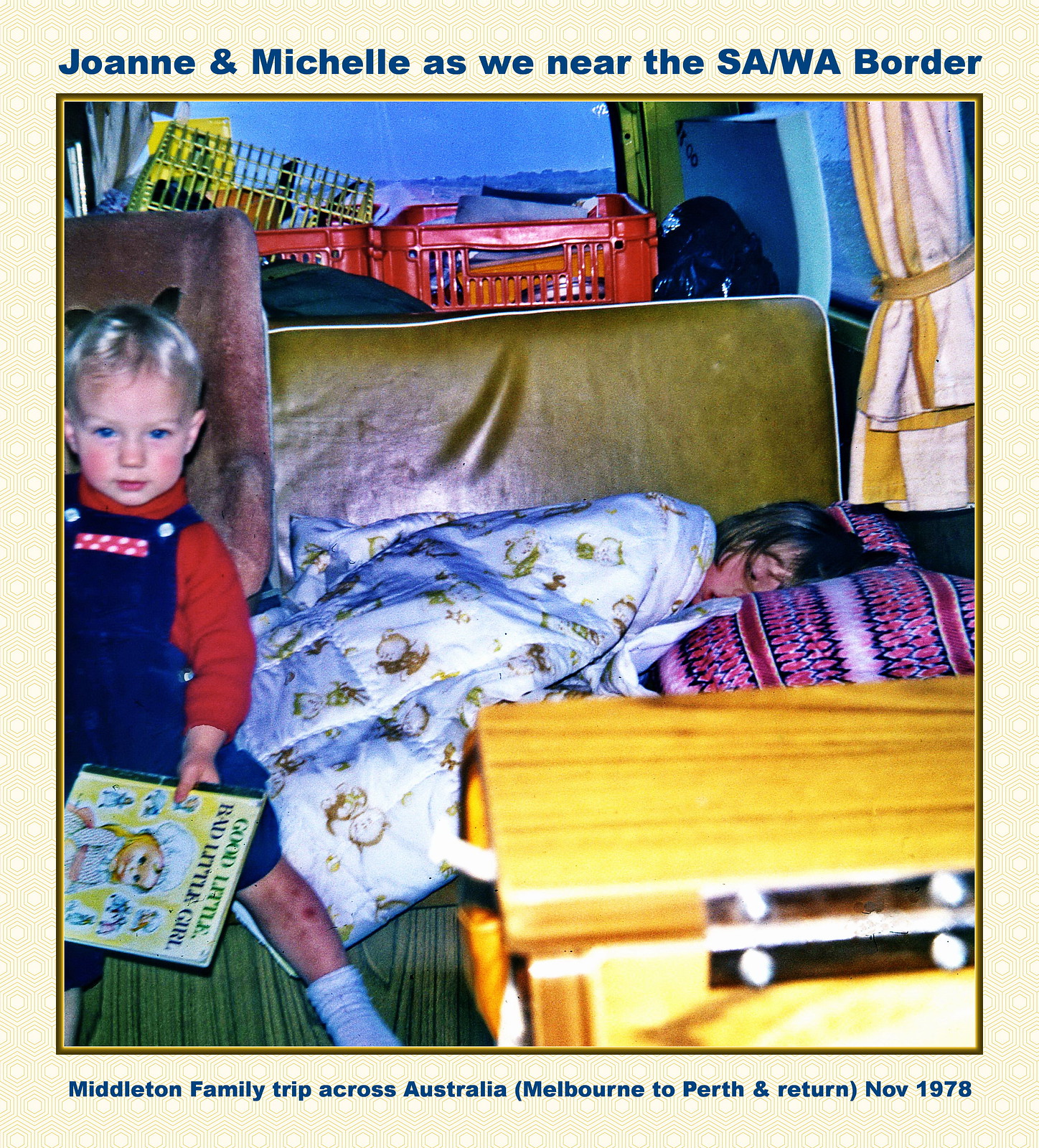This image is a square, old photograph with a light yellow, geometric-patterned border. At the top in navy blue text, it reads "Joanne and Michelle as we near the SA/WA border," and at the bottom in blue letters, it says, "Middleton family trip across Australia, Melbourne to Perth and return, November 1978." The picture depicts the backseat of a car or van. On the left, a young child with short blonde hair is wearing a red long-sleeve shirt, blue overalls, and white socks. The child is holding a book titled "Good Little Bad Little Girl." To the right, another child, presumably Joanne, is sleeping with her head on a red and pink striped pillow, covered with a white blanket decorated with small creatures. The car's interior features an olive-leather seat back, and the background shows red and yellow baskets, a trash bag, and a mountainous landscape visible through the windows. The scene captures a nostalgic moment from their family road trip in 1978.